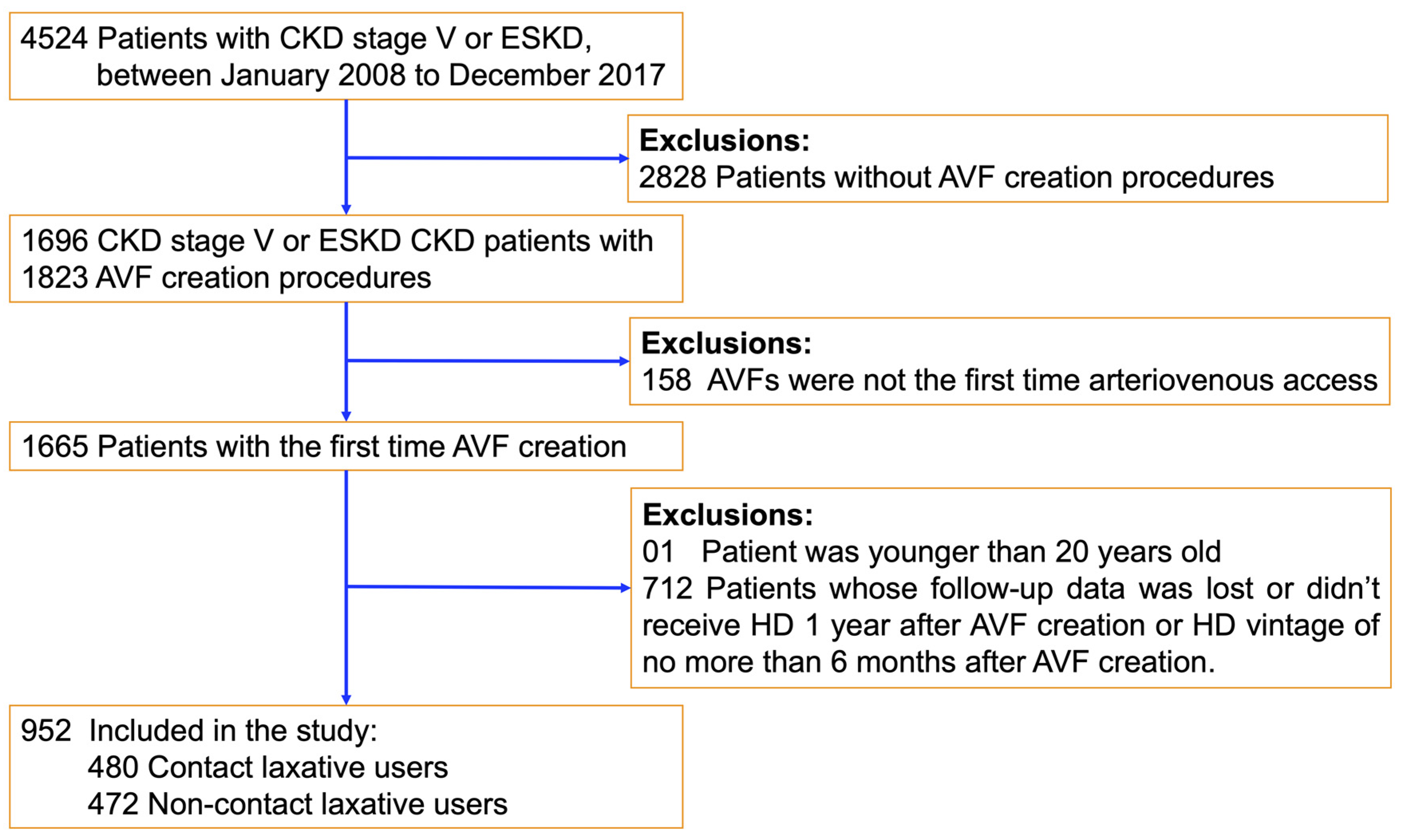The image depicts a flowchart of a scientific study involving the analysis of 4524 patients with Chronic Kidney Disease (CKD) Stage V or End-Stage Kidney Disease (ESKD) between January 2008 and December 2017. The chart details the progression and exclusion criteria of the study. Initially, 2828 patients without Arteriovenous Fistula (AVF) creation procedures were excluded. This left 1696 CKD Stage V or ESKD patients who had 1823 AVF creation procedures. An additional 158 patients were excluded because their AVF procedures were not the first-time access. Consequently, 1665 patients were identified as having first-time AVF creation procedures. Further exclusions included one patient younger than 20 years old and 712 patients due to lost follow-up data or insufficient hemodialysis (HD) history post-AVF creation. Ultimately, 952 patients were included in the study, divided into 480 contact laxative users and 472 non-contact laxative users. The diagram is visually represented with yellow-outlined boxes and blue arrows connecting each step of the study's criteria.